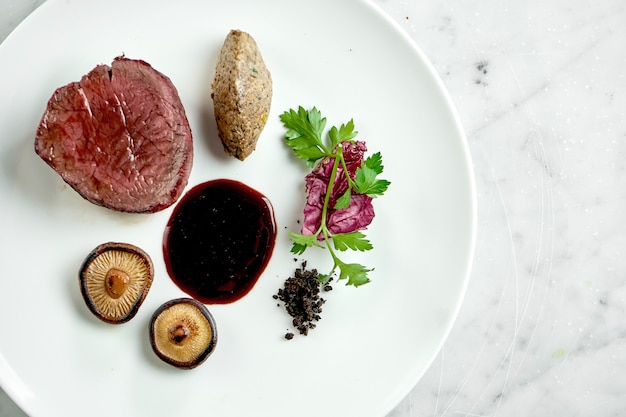This image showcases a fine-dining dish elegantly presented on a white plate set atop a white and gray marble table. The plate, partially cut off at the top and left edge, displays a nearly circular arrangement of rich brown demi-glace sauce at its center. The focal point is a filet mignon, cooked to a medium-rare with a vividly pink interior, positioned towards the upper left portion of the plate. Accompanying the steak are two upside-down chanterelle mushroom caps on the bottom left, the cut-off bases visible. Garnishing the dish are sprigs of green parsley, and dots of black peppercorns scattered beneath delicate celery leaves on the right side. Additionally, a hint of red cabbage and possibly foie gras adds to the sophisticated presentation, making it worthy of a high-end restaurant.